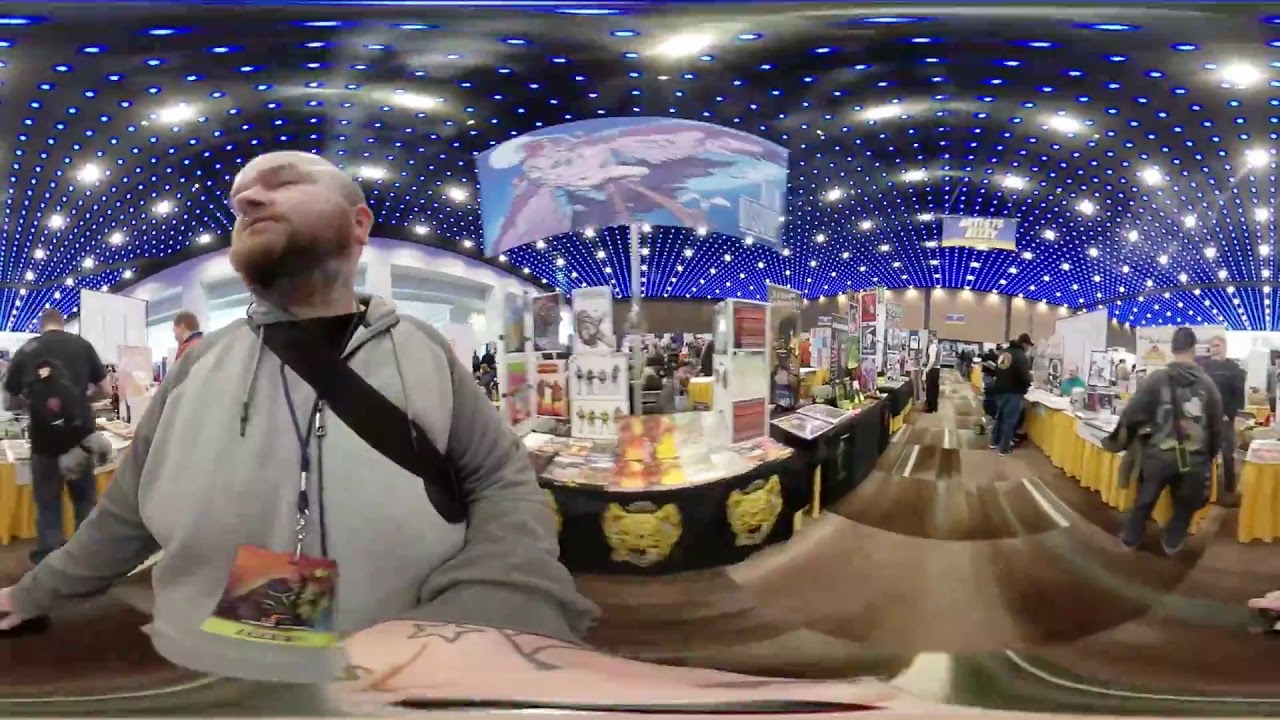This horizontal indoor photograph captures a bustling convention with various display booths and a crowd of attendees. The ceiling, an intricate geometric design marked by numerous small blue lights, contrasts against the gray backdrop with white spotlights. The ground is a blurred carpet with various shades of brown, populated by individuals navigating through tables and displays.

At the center of focus is a fair-skinned man with a goatee, a shaved head, and a notable black strap crossing his gray zip-up hoodie, likely for carrying a bag. He has a colorful badge hanging from a lanyard around his neck. His proximity to the camera makes his figure prominent, with his arm seemingly wrapped around the base of the camera lens.

The convention floor features several display booths: black-clothed tables with tiger emblems in the center, flanked by tables draped in yellow cloth on both the left and right. Brochures and informational materials are spread over the tables, inviting attendees to engage. In the distant background, video screens exhibit vibrant but indiscernible images, and the ceiling's constellation of blue and white lights adds a sparkling effect to the scene. Crowds of people traverse the aisles, stopping occasionally to interact with the displays and gather information.